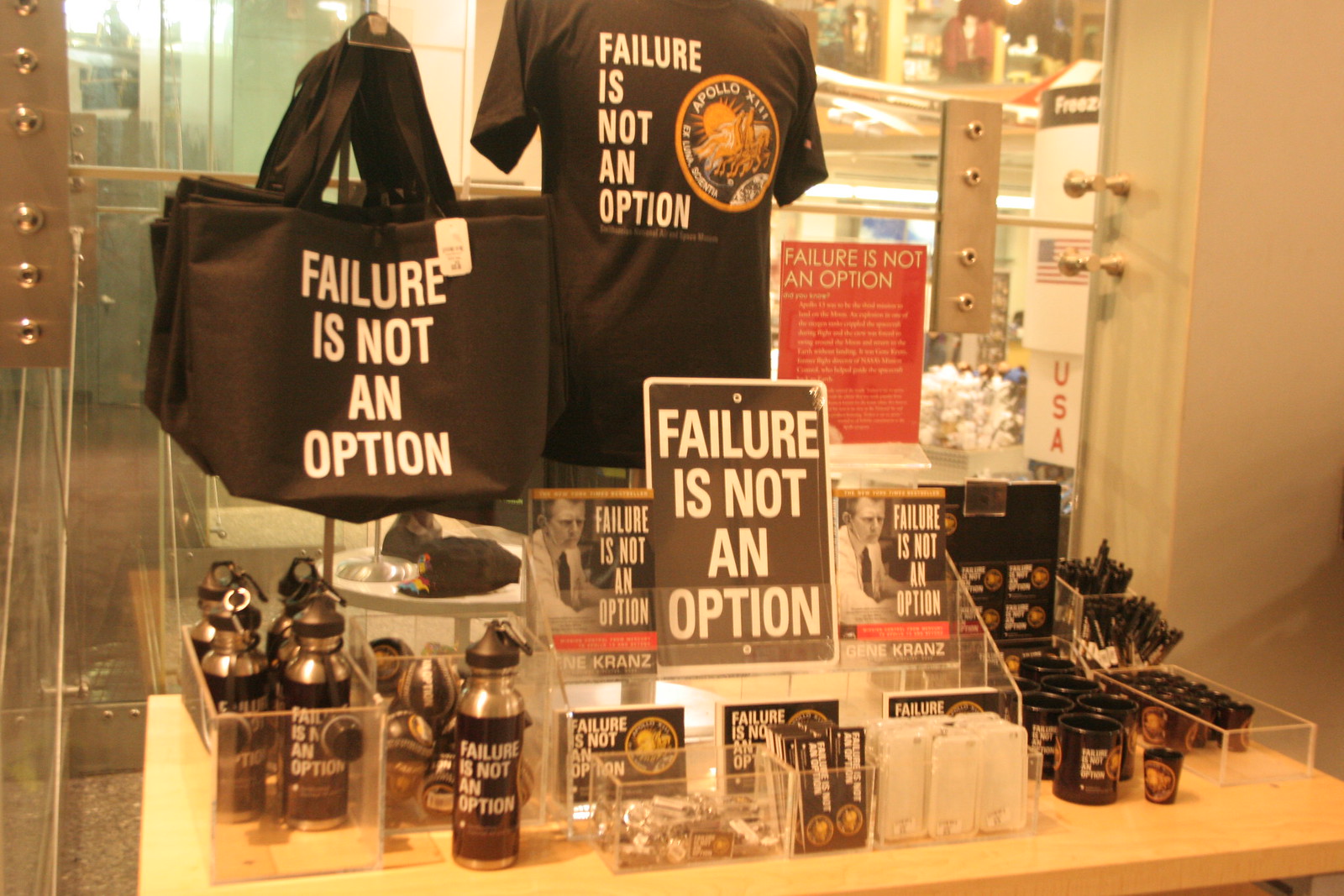The photograph showcases a detailed and organized product display centered around the motivational phrase "Failure is not an option." The display features a wide array of merchandise, all emblazoned with this slogan in white text on a black background. Key items include a black t-shirt featuring the Apollo 13 mission seal, black tote bags, a tin sign resembling a road sign, and a book by Gene Kranz titled "Failure is Not an Option." Additionally, the table holds water bottles, stress balls, keychains, cell phone cases, shot glasses, mugs, pens, and refrigerator magnets, all bearing the same inspiring message. 

The products are neatly arranged in clear bins on a light wooden table, and some items, like the t-shirt and tote bags, are hung for better visibility. An informational plaque provides context for the quote. The display is set against a backdrop with partially-visible text and an American flag sticker with "USA" in red below it. The photo itself is slightly blurry, with a yellowish hue, which affects the clarity and vibrancy of the colors.